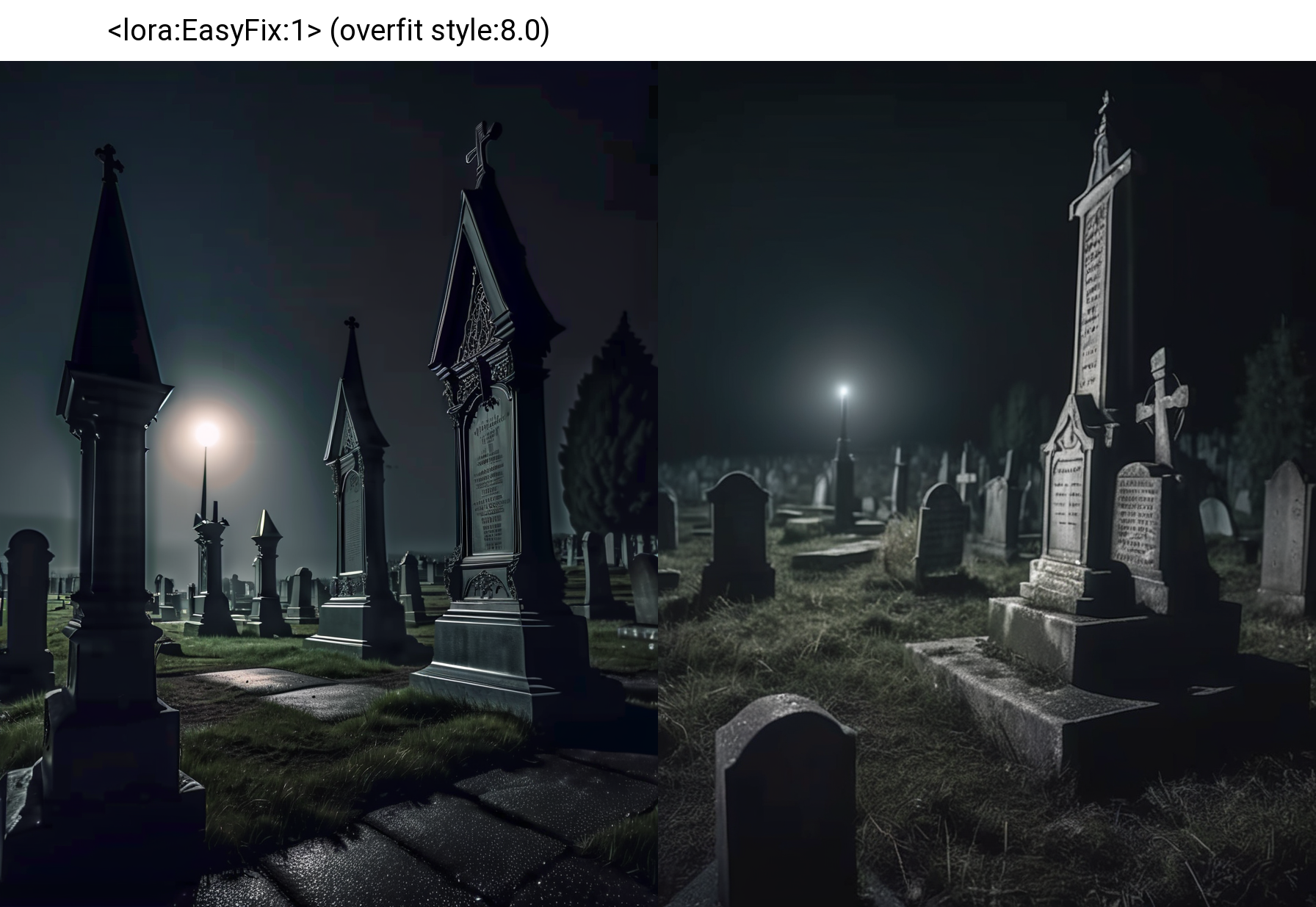This detailed image, likely a 3D rendering given the "Laura Easy Fix 1 Overfit Style 8.0" text at the top, is a composite of two graveyard scenes arranged side-by-side, forming a single, wider-than-tall rectangle. Both scenes depict a nighttime graveyard illuminated by a very bright light—possibly resembling a high-up streetlamp—against an otherwise black sky. The left image features a lush, green grassy area with headstones that have more intricate designs. Notably, there is a headstone resembling a grandfather clock with a cross on top, along with another similar headstone beside it. An evergreen tree is visible in the background.

In contrast, the right image displays a more barren, brown grassy area with conventional headstones, rectangular with rounded tops and one larger, more prominent headstone with extensive writing on it, also topped with a cross, resting on a pedestal. This side has a more minimalistic layout with fewer elaborate gravestones and appears to be from a different season due to the lack of greenery. Though the two images are distinct in their details and seasons, they share a similar atmospheric light source—a bright yellow or white light—adding a surreal and eerie illumination to the graveyards. The text above the image adds a clinical, AI-generated context to the dual graveyard scenes, enhancing their otherworldly and meticulously crafted nature.